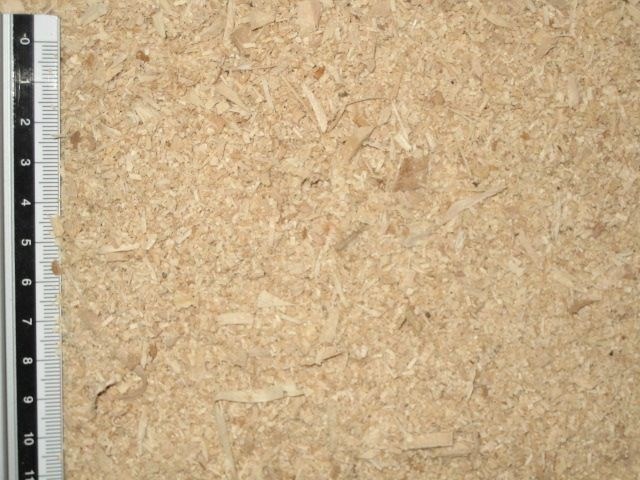In this image, a close-up shot depicts a light brown cork or particle board, distinguished by its rough texture and embedded dark fibers and wood fragments. The board, which appears dry and untouched by any damage, lies flat and ready to be measured. To the left side of the image, a white ruler with black measurement lines and a vertical black stripe displaying increments from 1 to 11 runs parallel to the board. The ruler's detailed markings help delineate inches and centimeters. This setup suggests preparations for a woodworking task, where precise measurements are crucial for cutting or assessing the board. The scene vividly conveys the practical, hands-on nature of the work being undertaken.